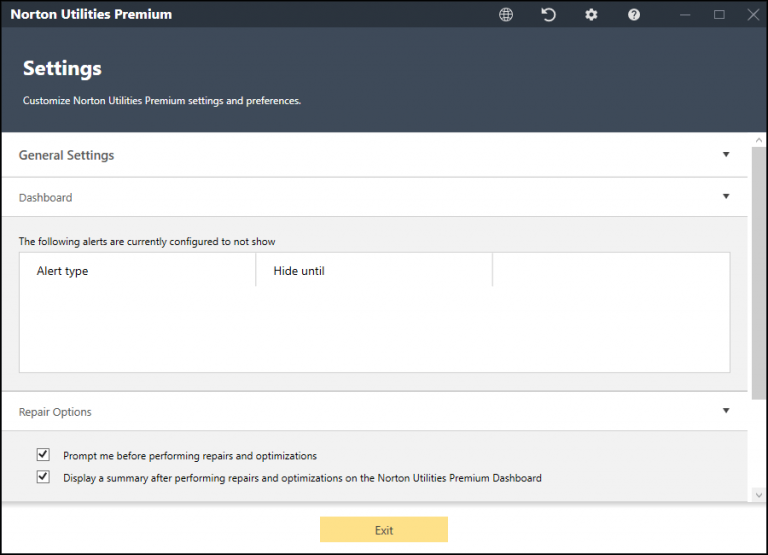In this image, a web page for Norton Utilities Premium is displayed. At the top of the page, a black header prominently features the Norton Utilities Premium branding. The header area of the screen, also dark grey or black, showcases the word "Settings" in large, white font, with "settings" repeated in smaller print beneath it, indicating the section for customizing Norton Utility Premium settings and preferences.

Below this header, the screen transitions to white, where it states "General settings" followed by a dropdown menu. Further down, another dropdown labeled "Dashboard" is visible. Moving downward, the text indicates "The following alerts are currently configured to not show" with columns titled "Alert Type" on the left and "Hide Until" on the right.

As we examine the page further, another dropdown for "Repair Options" is displayed. Below this dropdown, a checked box reads "Prompt me before repairs and optimizations," followed by another checked box stating "Display a summary after performing repairs and optimizations on the Norton Utilities Premium dashboard."